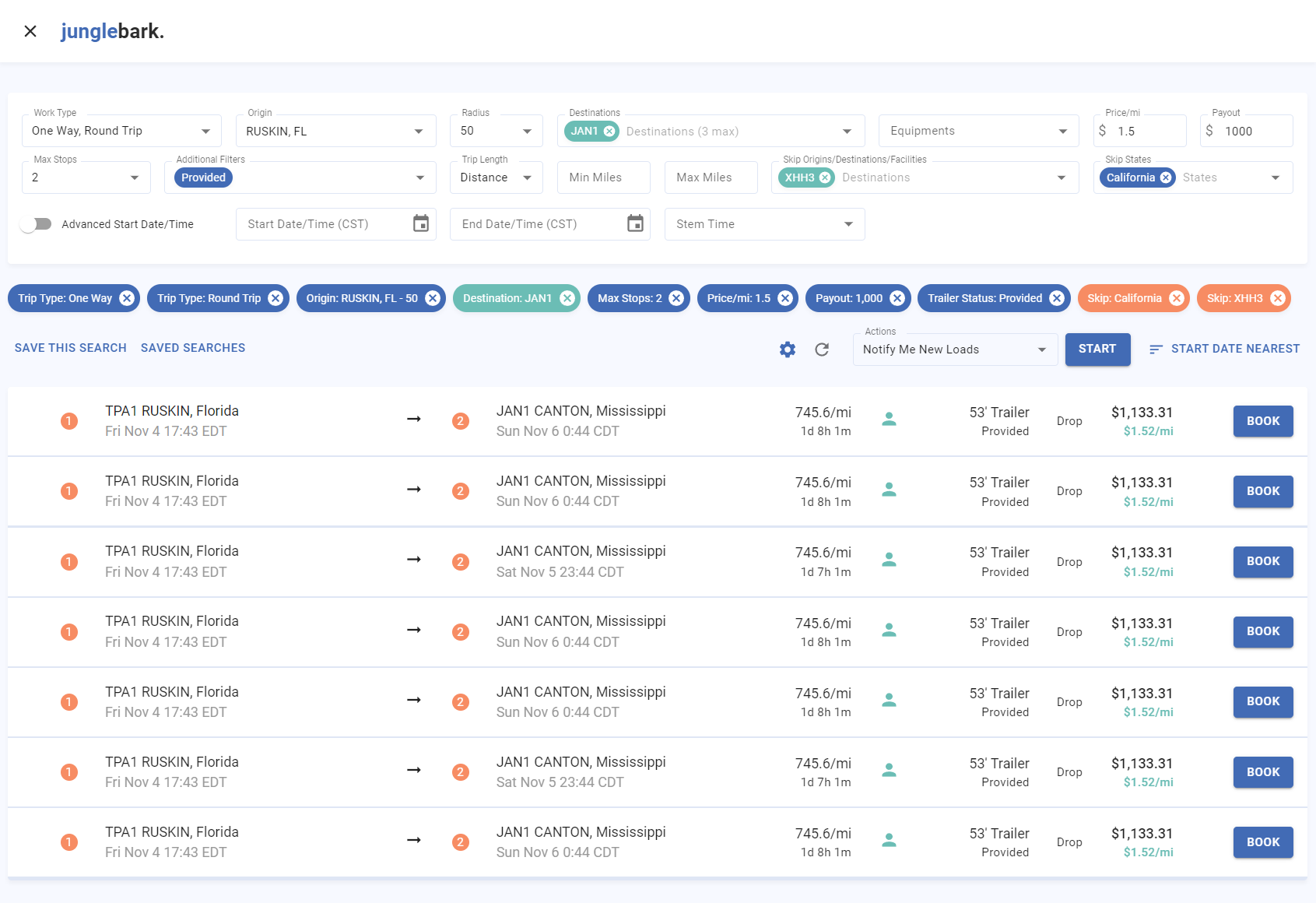The image features a website called "Jungle Bark," which appears to be a comprehensive travel or logistics platform. At the top of the site, several text fields invite users to input various details such as type of trip, origin, and destination. Users can specify if the trip is one-way or round-trip, although the text appears to be entered incorrectly. The origin is set to "Ruskin, Florida" with a 50-mile radius, and the departure or destination date is January 1st. 

The interface includes a list of possible transportation options, most likely aimed at truck drivers or logistics companies. Notably, it mentions the provision of a 53-foot trailer, indicating that the service caters to those needing to haul large quantities of goods. While the exact purpose of the site remains somewhat ambiguous, it strongly suggests a focus on logistics and transportation management for long-haul trucking.